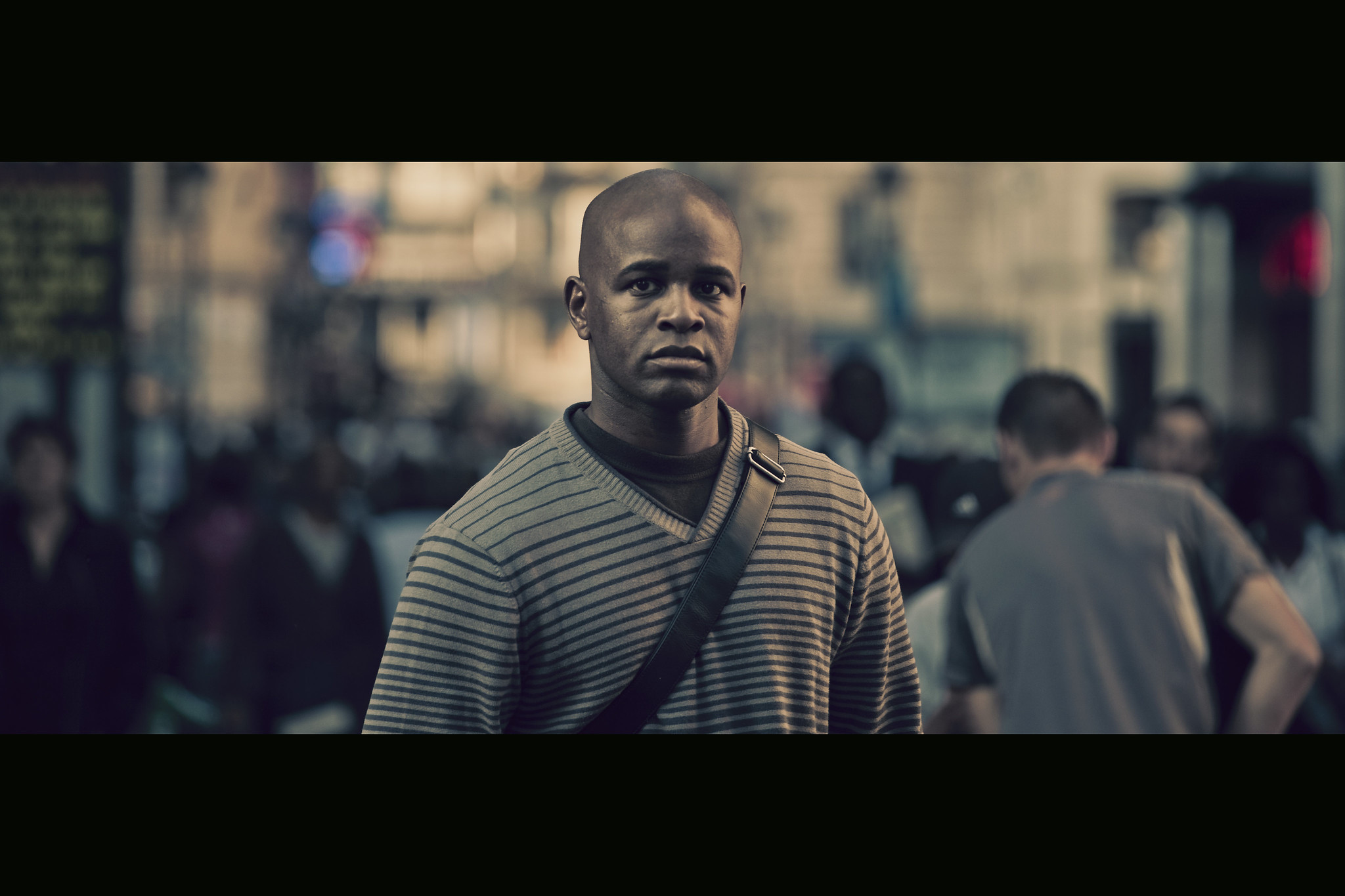The image features a young black man, likely in his 20s or early 30s, standing centered in the frame and facing forward, looking directly into the camera. He is bald and displays a solemn or neutral facial expression. He is dressed in a grey v-neck t-shirt with black stripes, underneath which he is wearing a black layer. Strapped across his shoulder is a black strap with a silver buckle, possibly part of a bag. The background is intentionally out of focus, adding a cinematic tone with slightly muted colors. Despite the blur, the scene appears to be a busy city street with crowds of people and buildings, emphasizing the isolation of the subject amidst urban hustle and bustle.